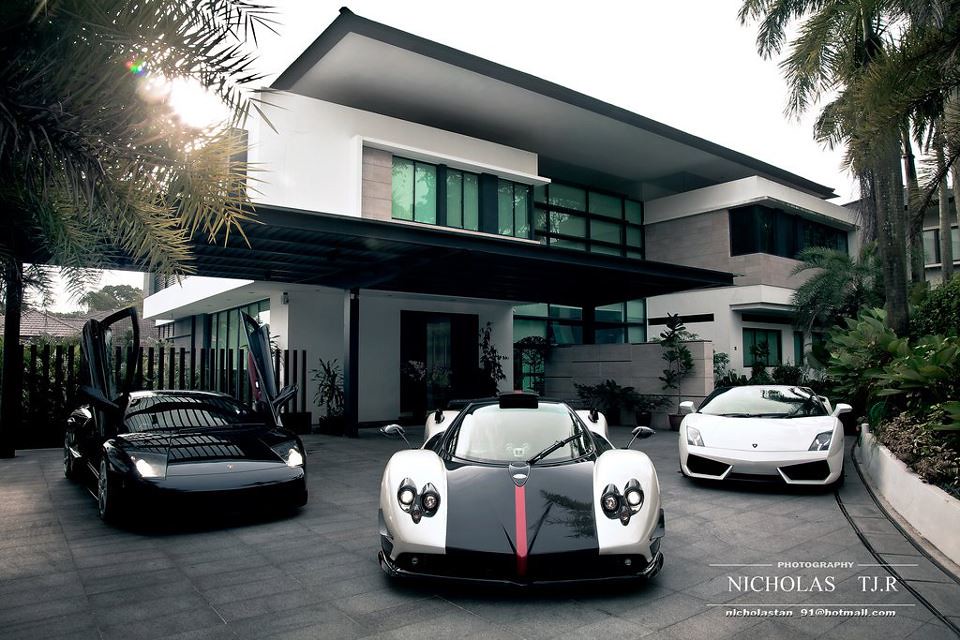This is a professional outdoor photograph showcasing a luxurious, modern two-story house with a flat roof and numerous glass windows. The house is predominantly white, reflecting the sunlight, which illuminates its sleek architectural design. A prominent feature on the top floor is a balcony with a row of pristine windows. On the first floor, some glass windows are intersected by a wooden fence extending from the left side of the image. In the foreground, a spacious tiled driveway hosts three high-end sports cars arranged in a semicircle. The leftmost car is a black model with winged doors open upwards, adding an element of grandeur. The centrally positioned car is a striking combination of white with a contrasting black stripe down the middle, accentuated by a vivid red line. The third car, also white, is located at the rightmost part of the driveway, positioned closer to the house. Complementing the scene, there is a touch of nature with palm trees framing the house on both the upper left and upper right corners, with one tree partially backlit by the sun. The bottom-right corner of the image features the photographer's mark: "Photography, Nicholas T.J.R."